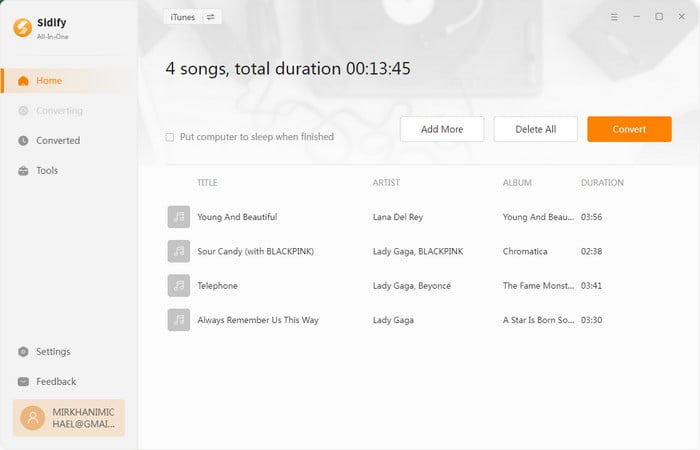This image, taken from the SIDIFY website, showcases a music conversion interface. Central to the display is the summary section, indicating four songs with a total duration of 13 minutes and 45 seconds. The end-of-process option "Put computer to sleep when finished" is notably present. In this section, there are clear buttons for "Add More," "Delete All," and a prominently orange "Convert" button, contrasting with the white buttons.

Below, the content is organized into four columns: Title, Artist, Album, and Duration. The song details are as follows:
1. **Title:** "Young and Beautiful"  
   **Artist:** Lana Del Rey  
   **Album:** Young and Beautiful  
   **Duration:** 3:56
2. **Title:** "Sour Candy"  
   **Artist:** Lady Gaga, Blackpink  
   **Album:** Chromatica  
   **Duration:** 2:38
3. **Title:** "Telephone"  
   **Artist:** Lady Gaga, Beyoncé  
   **Album:** (not specified)  
   **Duration:** unspecified
4. **Title:** "Always Remember Us This Way"  
   **Artist:** Lady Gaga  
   **Album:** (not specified)  
   **Duration:** unspecified

This detailed layout provides a comprehensive overview of the tracks queued for conversion.